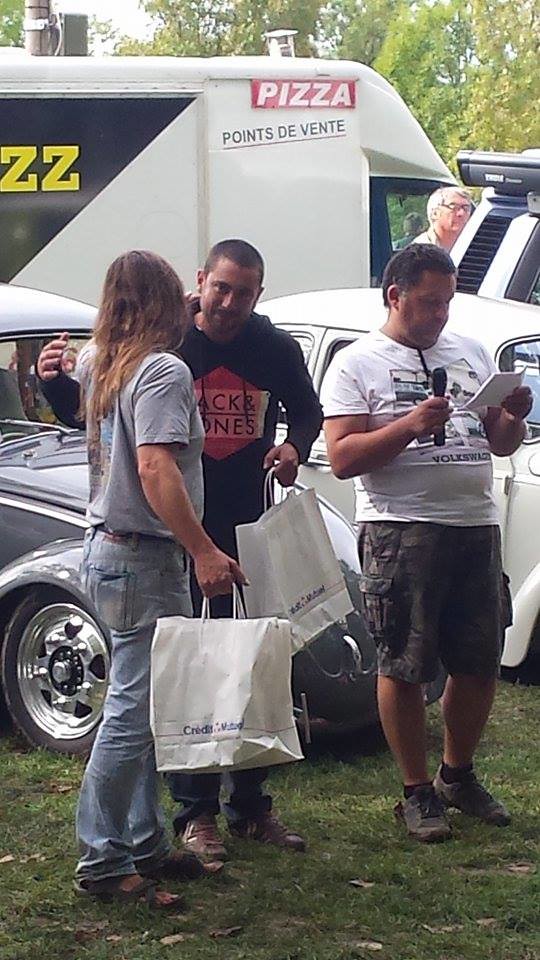The photograph captures a lively scene at a car event with multiple people in an outdoor setting. In the foreground, three men are prominently featured. On the left, a man with long blonde hair cascading below his shoulders is wearing open-toed sandals, blue jeans, a brown belt, and a short-sleeve graphic t-shirt. He holds a white paper bag with a blue "Credit Mutual" logo by its white handles. Beside him, another man, sporting a blue pullover hoodie with a "Jack and Jones" diamond logo, brown shoes, and blue jeans, also clutches a similar white "Credit Mutual" bag. The two men are semi-embracing each other with one arm each. To their right, the third man, with short dark hair, is dressed in a white t-shirt adorned with a central graphic, camouflage shorts, and black shoes. He speaks into a microphone while reading from a piece of paper. In the background, various cars and a large van bearing the word "Pizza" in white letters on a red background are visible against a backdrop of green trees and grass, emphasizing the open, vibrant space of the event.